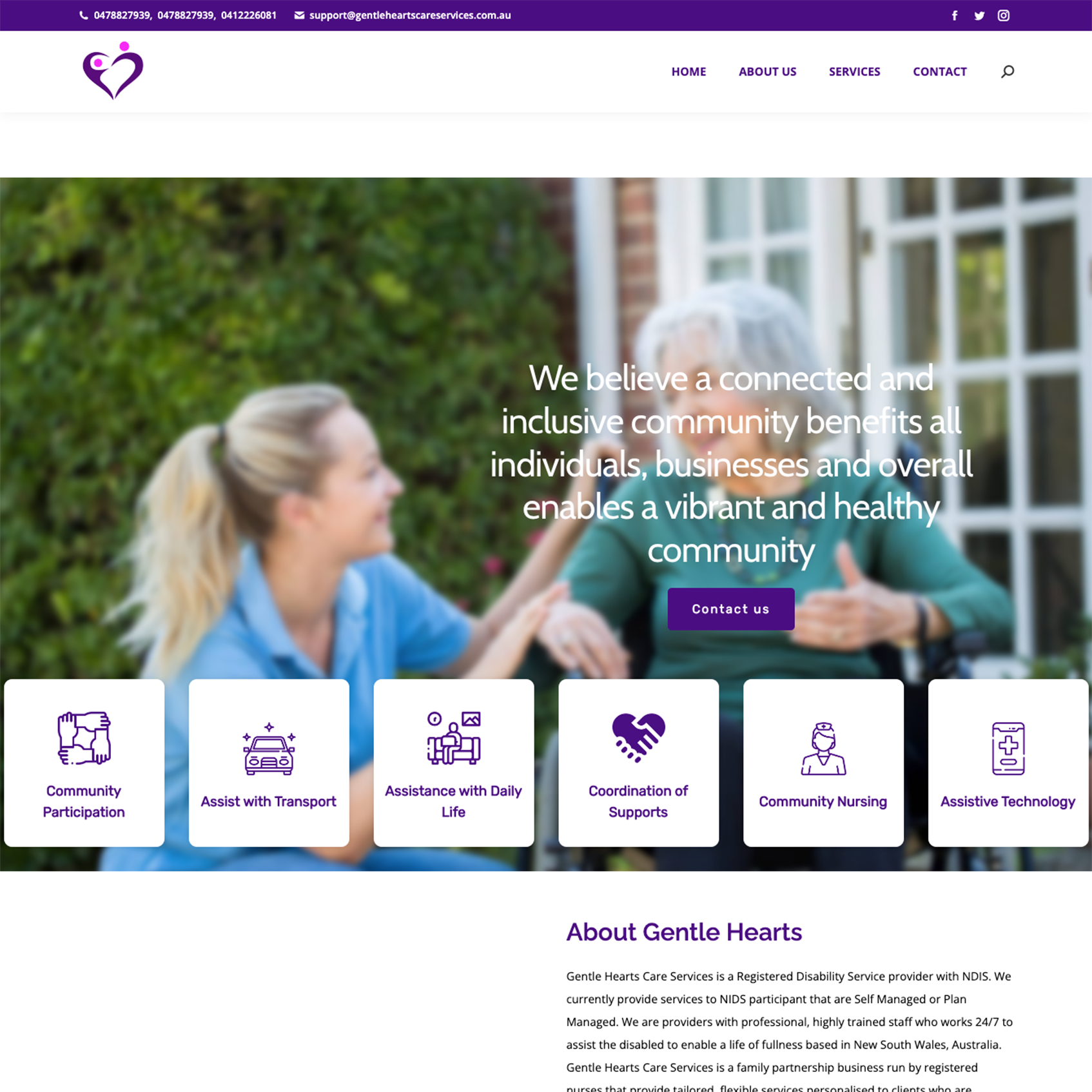The image is a left-to-right horizontal screenshot of a website that can be accessed on a computer or smart device. The background predominantly features a white area from the computer screen. At the top of the image, there is a slim, long, purple rectangular bar that includes a phone icon with a phone number on the upper left-hand corner, followed by an email icon with an email address. The banner indicates an Australian location and displays clickable social media icons for Facebook, Twitter, and Instagram.

On the left side of the white background, there is a small heart graphic accompanied by a couple of pink circles. To the upper right, the website features navigation options labeled Home, About Us, Services, Contact, and a magnifying glass icon for search functionality. 

The main content includes a slightly blurred image depicting a woman conversing with an elderly woman who is seated in a wheelchair. The backdrop consists of trees and a building with visible windows. Superimposed text over the image reads, "We believe a connected and inclusive community benefits all individuals, businesses, and overall enables a vibrant and healthy community." 

Below the image, a purple "Contact Us" button is prominently displayed. At the bottom of the screen, there are white square buttons with various icons and labels, including Community Participation, Assist with Transport, Assistance with Daily Life, Coordination of Supports, Community Nursing, and Assistive Technology. The footer contains a brief description about Gentle Hearts.